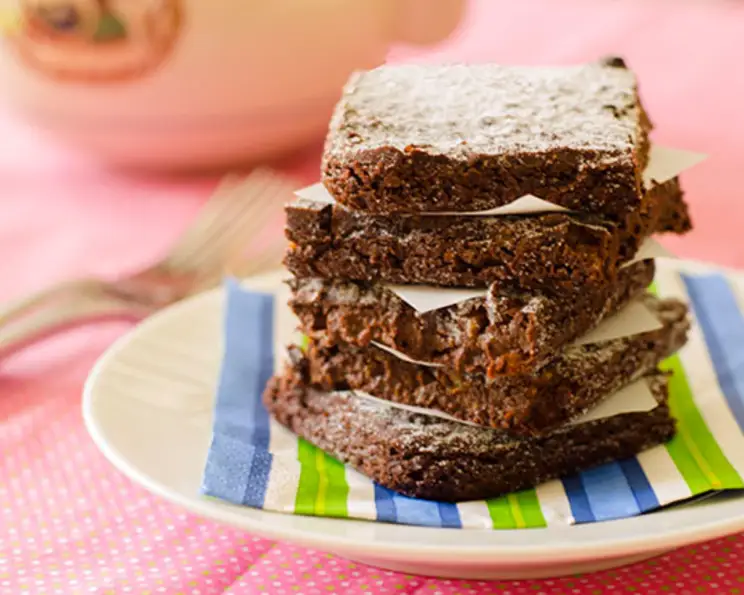In the photograph, a stack of five small dessert bars, possibly brownies, are meticulously arranged on a white circular plate placed center stage. These brownies, each approximately 2x2 inches in size and less than half an inch in height, are liberally dusted with powdered sugar. Separating each layer is a piece of what appears to be white parchment or baking paper. The plate itself sits atop a vibrant napkin adorned with blue, white, lime green, and yellow stripes, adding a splash of color to the presentation. This setup rests on a pink tablecloth adorned with tiny white and yellow polka dots. To the left side of the frame, there is a gold-colored fork positioned near the plate, and two silver forks can also be seen. Additionally, the upper left corner of the image features what appears to be a piece of orange pottery, contributing to the overall warmth and homeliness of the scene.